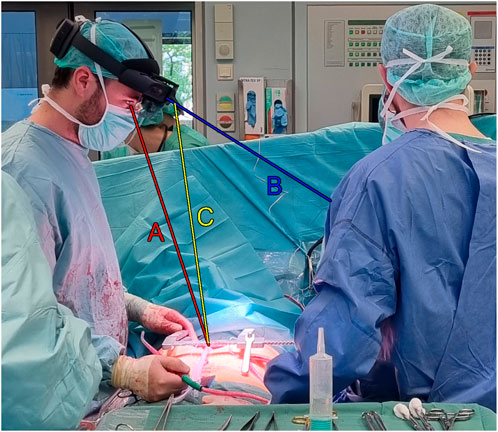In a bustling operating room, three medical professionals focus intently on a surgical procedure. The main surgeon, positioned on the left, is identifiable by his blood-splattered medical smock and advanced headgear, which includes goggles with lights, perched on his forehead. His attire, in light blue, matches the surgical standards. From his location, a red line labeled "A" extends downward, indicating his line of sight to the operating area. Nearby, a second doctor, with their back to the camera, is clad in darker blue scrubs and protective headwear. A yellow line labeled "C" traces the path from the first surgeon’s visor to the surgical site, highlighting another visual angle. A blue line labeled "B" stretches towards this second doctor, possibly linking communication or focus points. In the background, just a glimpse of a third medical staff member's neck is visible, denoting a supportive role. The setting is further detailed by a tray laden with essential surgical tools, including scissors, tweezers, a syringe, and a plastic squirt bottle, positioned within the fore area of the image. The sterile white walls in the background, adorned with glove dispensers, further establish the clinical environment.